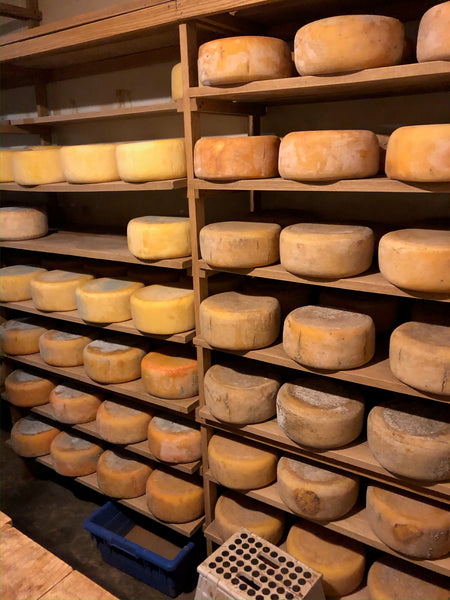This portrait-oriented color photograph captures the interior view of a cheese storage room, organized with shelves filled from floor to ceiling with round cheese wheels, also referred to as cheese hoops. These cheese wheels, varying in hue from bright yellow to deep brown, are meticulously arranged by type across two vertical columns of shelving. Each shelf in the left column typically holds four cheeses, except the third shelf down, which uniquely features only two cheeses spaced apart. The section on the right is entirely filled with cheese wheels, while the left section has the top shelf empty, revealing a blue container neatly tucked underneath. At the bottom of the image, a white step stool with black dot perforations, possibly made of steel, is stationed below the shelves, accompanied by some visible wood planks on the bottom left. The cheeses on the shelves appear moldy and dusky, enhancing the scene’s authentic aged ambiance reflected in the photograph's realistic, representational style.